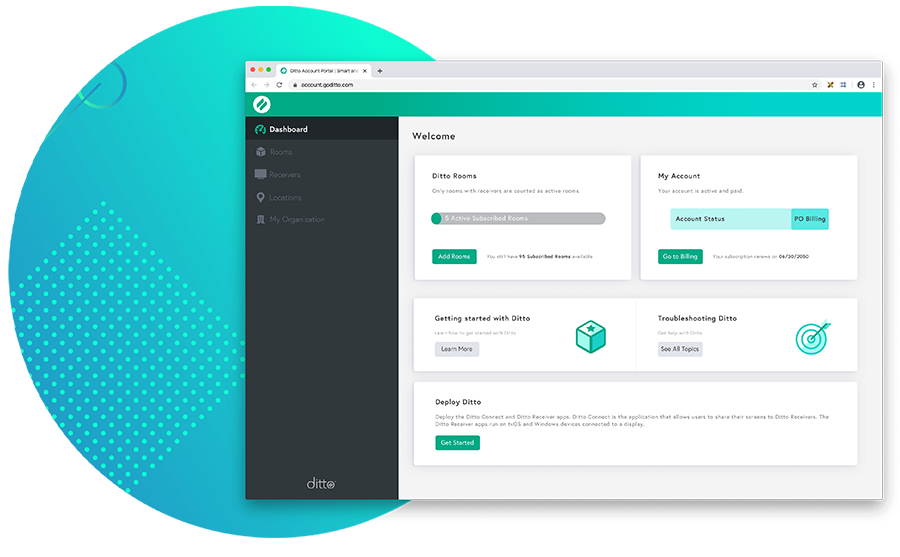The image depicts a user interface with distinct sections and detailed elements. On the left side, there's a large circle, primarily blue with a greenish tint on the right, filled with tiny dots. Adjacent to this is a square area composed of small blue dots, and at the top left of this section, there's a semicircular indent with a tiny blue line.

The interface showcases a web page with a gray background and two tabs; one features a green circle, the other a small gray circle. Below this, a long green strip includes a white circle with two green lines.

To the left, a dashboard with a black background and white text is visible, featuring a green semicircle and four icons underneath. The right section of the interface has a light blue background, with "Welcome" at the top, followed by "Ditto Rooms". Below this, there's a gray bar with a green circle at the start, and a green “Add Room” button at the bottom.

The "My Account" section contains a blue box labeled "Account Status" and a darker blue box marked "P.O. Billing" with a green “Go to Billing” button. Another white box titled "Getting Started with Ditto" has a gray “Learn More” button. The "Troubleshooting Ditto" section features a green square with a star, a dartboard icon with a dart, and a gray “See All Topics” button. Lastly, the "Display Ditto" section has a green “Get Started” button.